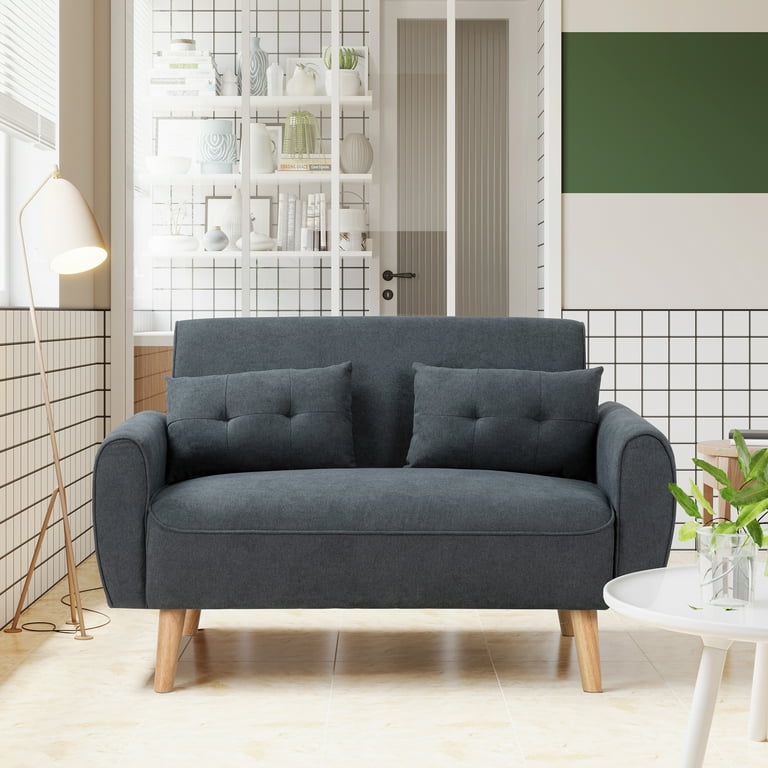In a well-lit, minimalist living room, the focal point is a sleek, mid-century gray loveseat featuring tufted back cushions with two buttons and slim, light wooden legs. Adjacent to the loveseat on the left side, a standing lamp with a tripod base casts a warm glow, its cord trailing discreetly behind the couch. To the right, a small, white and brown coffee table is adorned with a vase containing a lush plant, adding a touch of nature to the scene. The room's aesthetic is further enhanced by a backdrop of crisp white walls divided into a grid by thin black lines, lending a modern, structured feel. Behind the couch, white shelving units display an array of books, vases, and other decorative items, contributing to the room's clean and organized appearance. A glass door in the background offers a glimpse into a small office space, maintaining the overall theme of stark white with elements of natural wood and greenery.